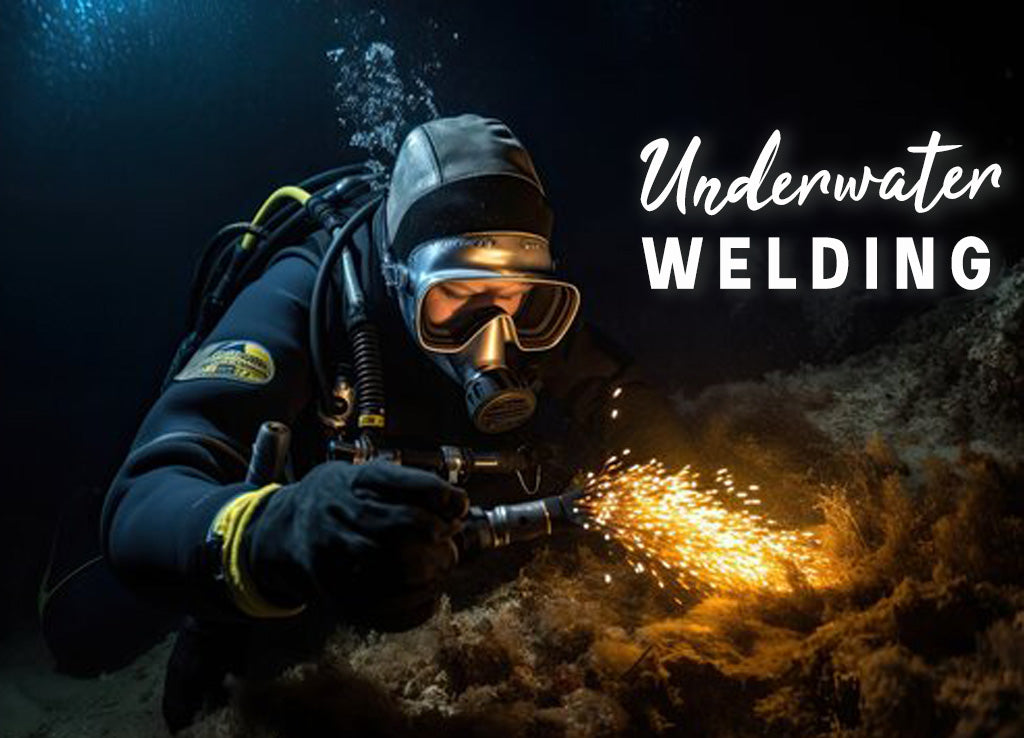The image depicts an underwater scene with a predominantly dark blue background. A person, identifiable by their white skin but not their gender, is central to the photograph. They are geared up in a black scuba diving outfit with yellow trim and are wearing black gloves. Over their head is an extended hood, and they have large, chrome-colored goggles. The scuba mask features a black stripe and an oxygen apparatus with a black tip, connected to black and yellow hoses that trail behind them, feeding into a tank on their back.

This individual is engaging in underwater welding, holding a welding tool in their right hand. Bright sparks emanate from the tool, providing a stark contrast to the surrounding darkness. Bubbles rise from their equipment, adding to the underwater ambiance. The top left corner of the image shows a faint beam of light shining through the water, while the bottom right corner includes some sea moss and other underwater elements. On the right side of the image, the words "Underwater" in cursive script and "WELDING" in bold capital letters are noticeable.